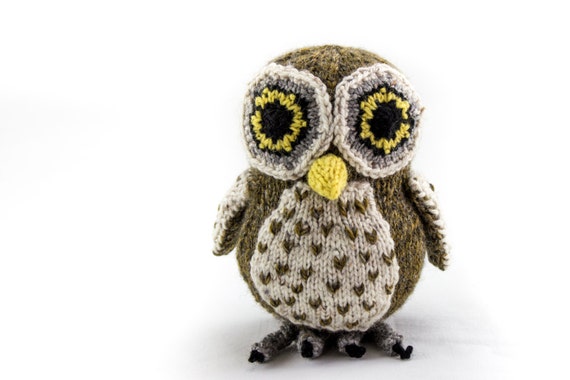The photo features a meticulously crafted crochet owl plushie, displayed against a solid white background that prominently highlights the shadow cast by the toy. The owl has a charming, cutesy appearance with a detailed design. Its body is predominantly brown, with a contrasting white belly adorned with brown triangle patterns. It features grey feet and wings that match the grey circles around its eyes. The owl's eyes are intricately detailed, composed of four concentric circles: a white outer edge, followed by grey, black, and yellow, with a black pupil at the center. The beak is a vivid yellow, adding a colorful touch to the otherwise neutral palette. Overall, this handcrafted owl plushie is an exquisite combination of textures and colors, presented on a clean, white surface.